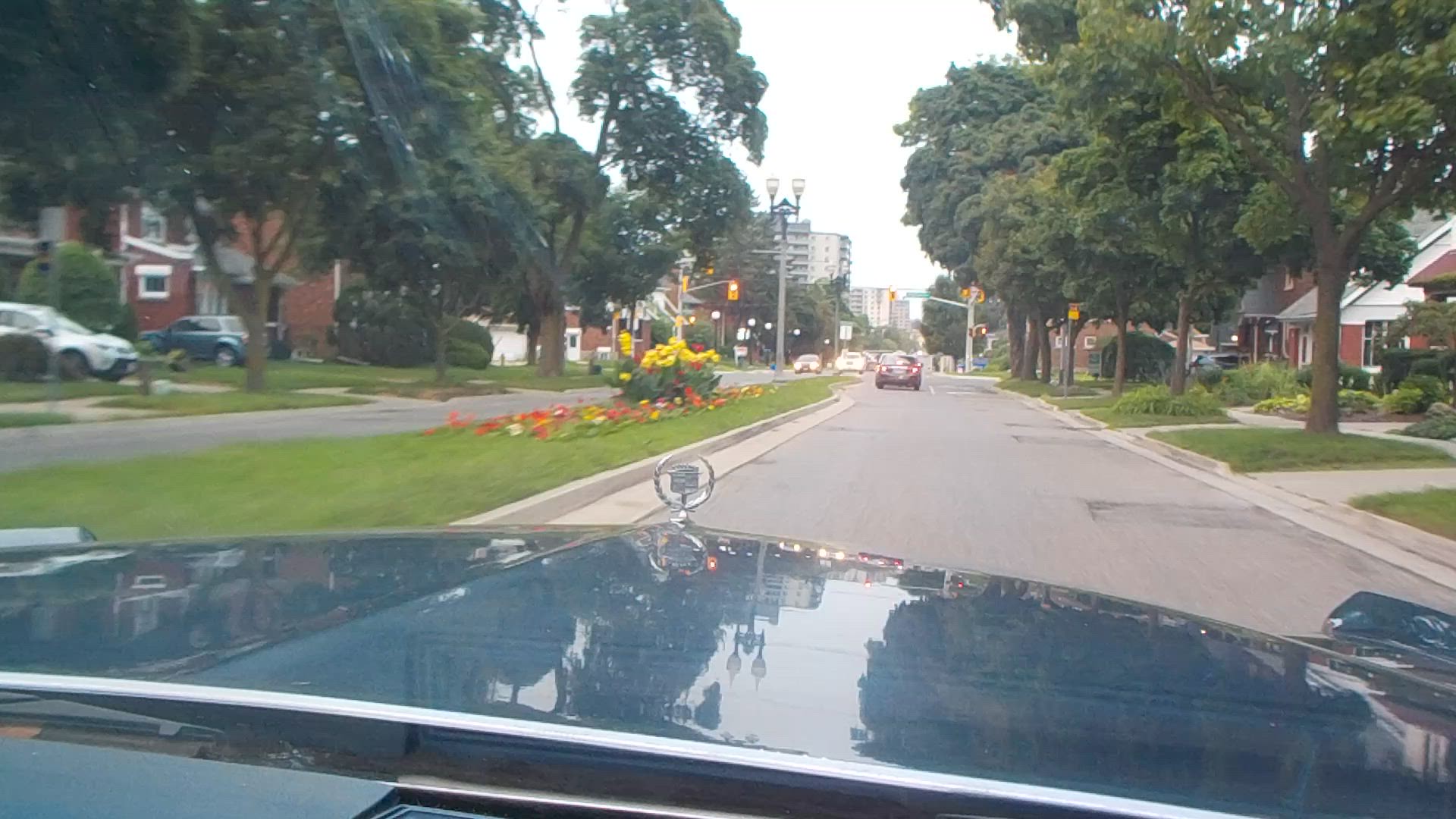The photograph, taken from inside a car, offers a view through the windshield. The hood of the car visible in the foreground is a vibrant blue, characterized by a central ridge and an emblem at the front featuring two small silver half-circles extending from its sides. Stretching ahead, the road is a mundane shade of gray. A red car can be spotted in the distance before a traffic light. On the right side of the image, plots of well-kept grass are bordered by sidewalks that lead inward. Meanwhile, the median strip to the left is lined with lush green grass adorned with clusters of red and yellow flowers. Beyond this median lies another gray road. Flanking this secondary road are residential houses, each with driveways home to a couple of parked cars: a white one in one driveway and a blue one in another. Tall, bushy green trees frame the scene on both sides. In the far left background, a tall building and a potential cell phone tower are also visible, adding a touch of urban silhouette to the suburban landscape.